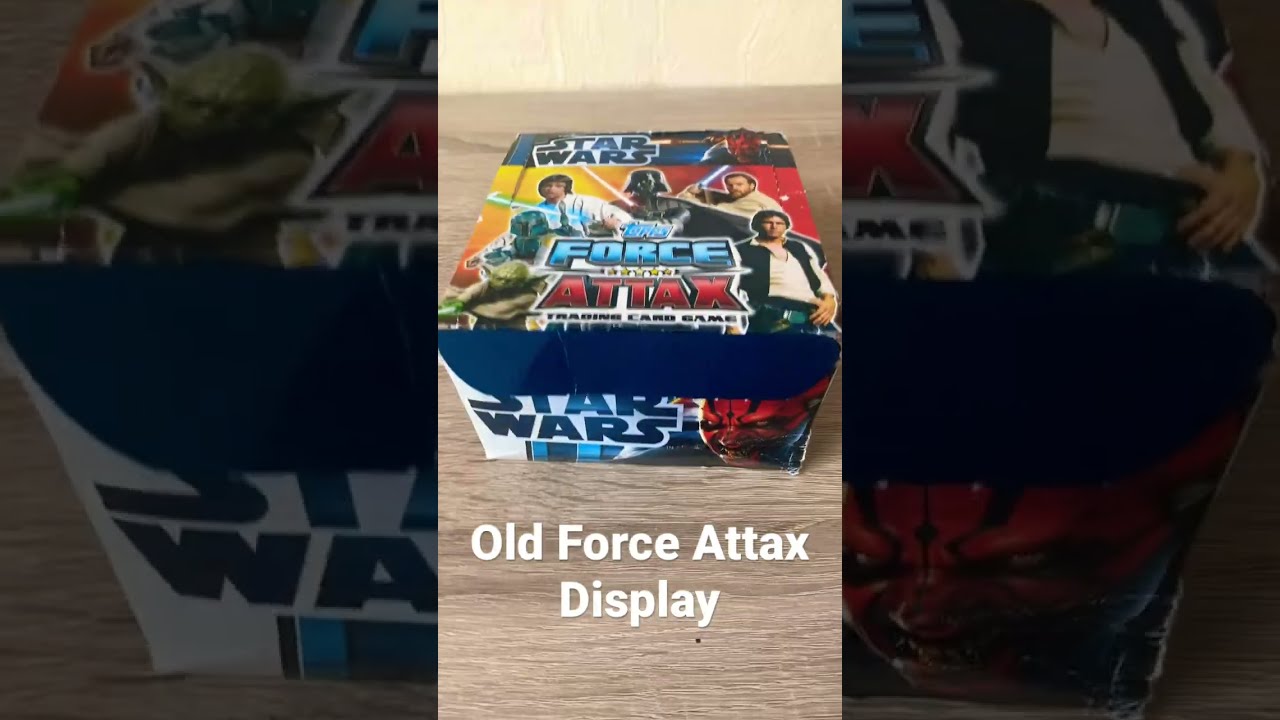The photograph showcases a Star Wars box, seemingly aimed for sale, positioned on a light-colored faux wood patterned floor against a beige wall backdrop. This rectangular box centers an image framed by a zoomed-in version of the same image, adding a visually arresting overlay. The top left corner of the box prominently displays the "Star Wars" logo. Illustrated on the cover are various iconic characters meticulously positioned: Yoda on the bottom left, Boba Fett above Yoda, Luke Skywalker above Boba Fett, with Darth Vader to the right of Luke. Further right is Ewan McGregor's portrayal of Obi-Wan Kenobi, and below him, Harrison Ford’s Han Solo. Dominating the box’s foreground is a strikingly red-faced depiction of Darth Maul. Central to the image, it reads "Topps Force Attax Trading Card Game," echoed by "Old Force Attax Display" on the lower portion. The background hues transition through dark tones with highlights of yellow and red, symbolizing the dichotomy of the light side and dark side.